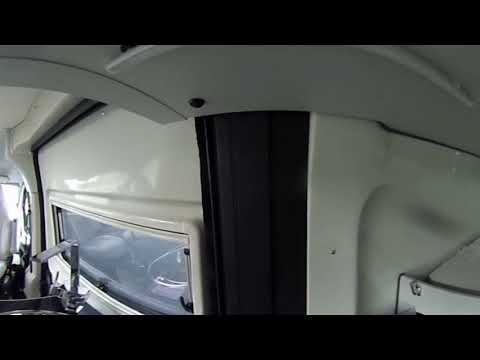The photograph captures a zoomed-in view of the interior of what appears to be a train, characterized by its smooth, white plasticky walls and a ceiling that resembles an overhead storage compartment. On the bottom left corner, there is a long, narrow rectangular window with a black handle on the right side. The image also features a strip of black material running vertically, which is possibly a curtain or part of the vehicle's structure. The setting is illuminated, but the overall photo is blurry, preventing a clear view through the window, which shows only a greenish blur. The scene contains no people or text, focusing solely on the vehicle's constructed elements, including metal sections with visible rivets.